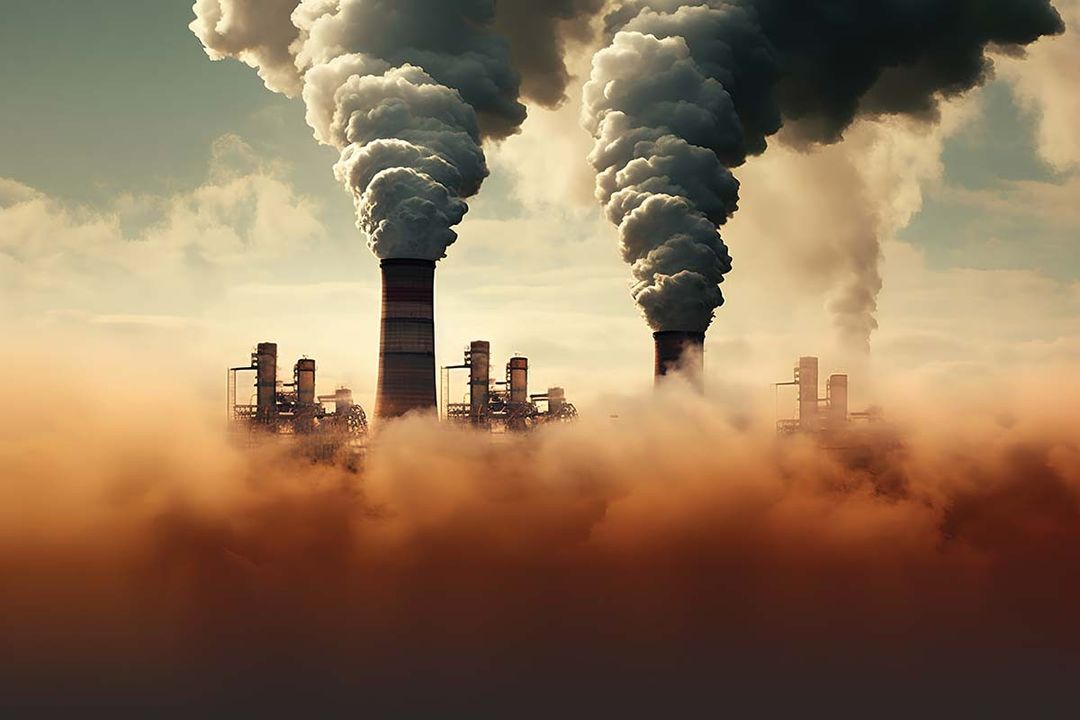The image depicts an AI-generated scene of an industrial power plant, possibly nuclear or coal-powered, featuring two massive, silo-sized smokestacks ejecting voluminous amounts of thick black smoke into the sky. The foreground is suffused with a brownish, smoggy mist that partially obscures the view of the factory buildings, which appear in light bronze or brown tones. The atmosphere around the plant is heavily polluted, with clouds of orange, red, and burgundy mingling with the dense smoke, creating an almost captivating yet ominous visual effect. In the background, additional chimneys and machinery are visible, contributing more smoke and steam to the already murky environment. Despite the overwhelming pollution, patches of clear blue sky can be seen above the factory, contrasting sharply with the otherwise muddy and murky surroundings.